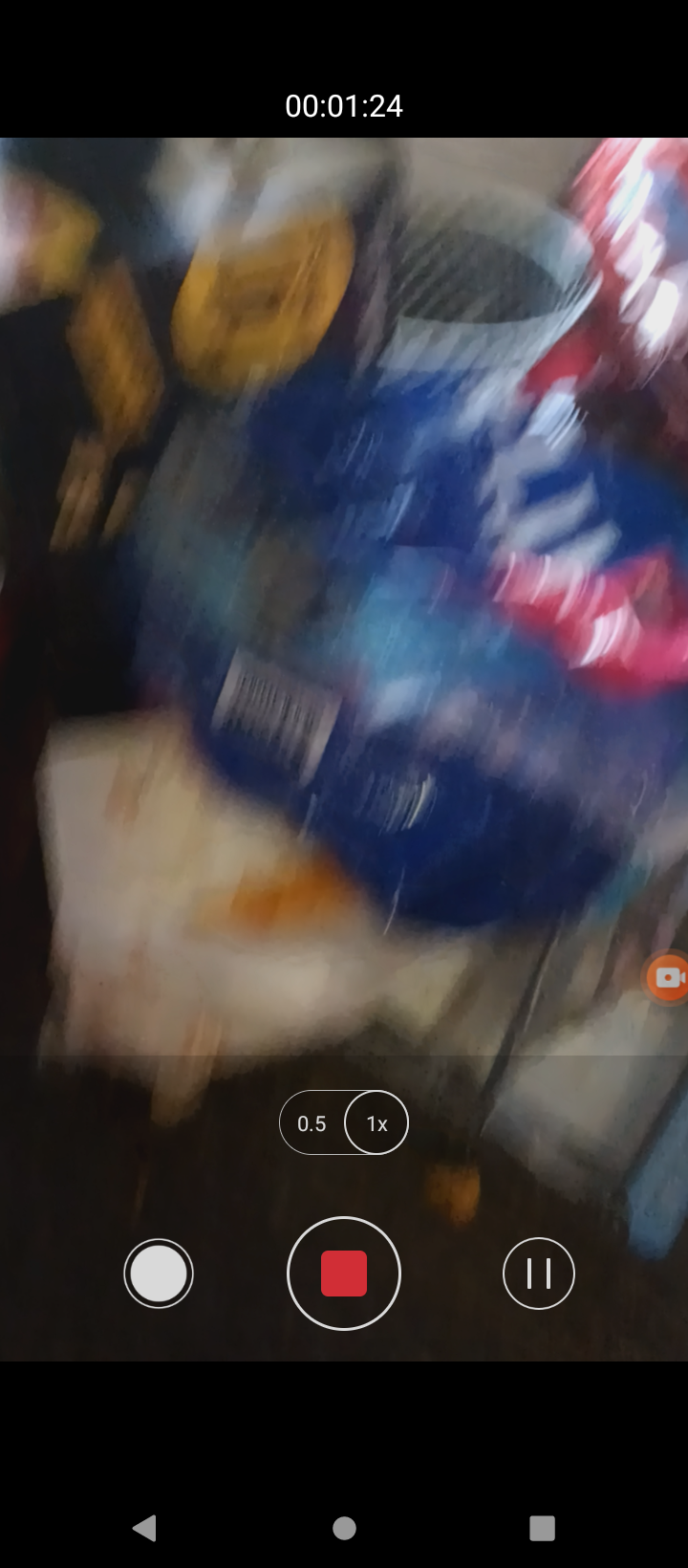This image appears to be a screenshot taken from a smartphone during the recording of a video. The screen is dominated by an extremely blurry image in which it's difficult to discern specific objects, though there are hints of a table with a metallic leg, possibly accompanied by a blue and red plastic bag, and perhaps a counter with some items on it. The background might feature a curtain with sunlight shining through, but it's very indistinct.

At the top of the screen, a black bar displays a timestamp, indicating the recording has been going on for approximately 1 minute and 24 seconds. The lower part of the screen features several controls: a '0.5x' zoom indicator, a button with a cross, a white circle containing a red square (indicating the recording is in progress), and another white circle with two lines, likely a pause button. Additionally, there's a video record icon positioned towards the bottom right. The overall scene is chaotic due to the severe blurriness, making it impossible to definitively identify the setting or the objects within the image.